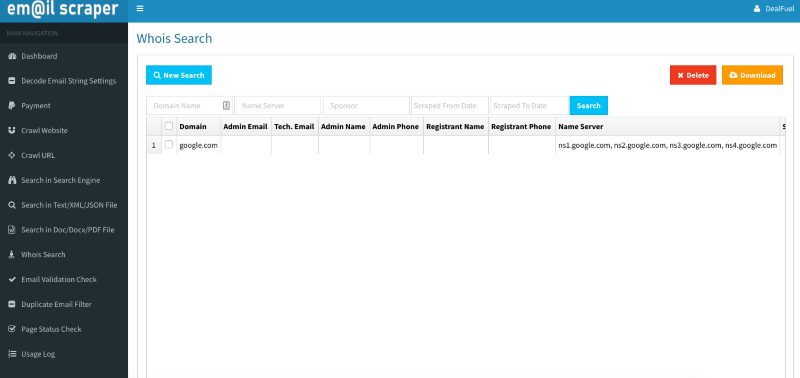This image is a detailed screenshot of an online tool called "Email Scraper." In the top left corner, the Email Scraper logo is prominently displayed, featuring the text "Email Scraper" with the 'A' in "email" replaced by an '@' symbol. 

Beneath the logo, the left column of the screen houses the primary navigation menu, set against a black background. This menu lists various options in the following order: Dashboard, Decode Email String Settings, Payment, Crawl Website, Crawl URL, Search in Search Engine, Search in Text/XML/JSON File, Search in Doc/DocX/PDF File, WhoIs Search, Email Validation Check, Duplicate Email Filter, Page Status Check, and Usage Log.

The main area of the page is currently focused on the "WhoIs Search" feature, as indicated by the title at the top of this section. Directly underneath this title, there is a button labeled "New Search." A chart occupies the majority of this space, with "Google.com" listed under the domain column, likely depicting the result of a previous search query.